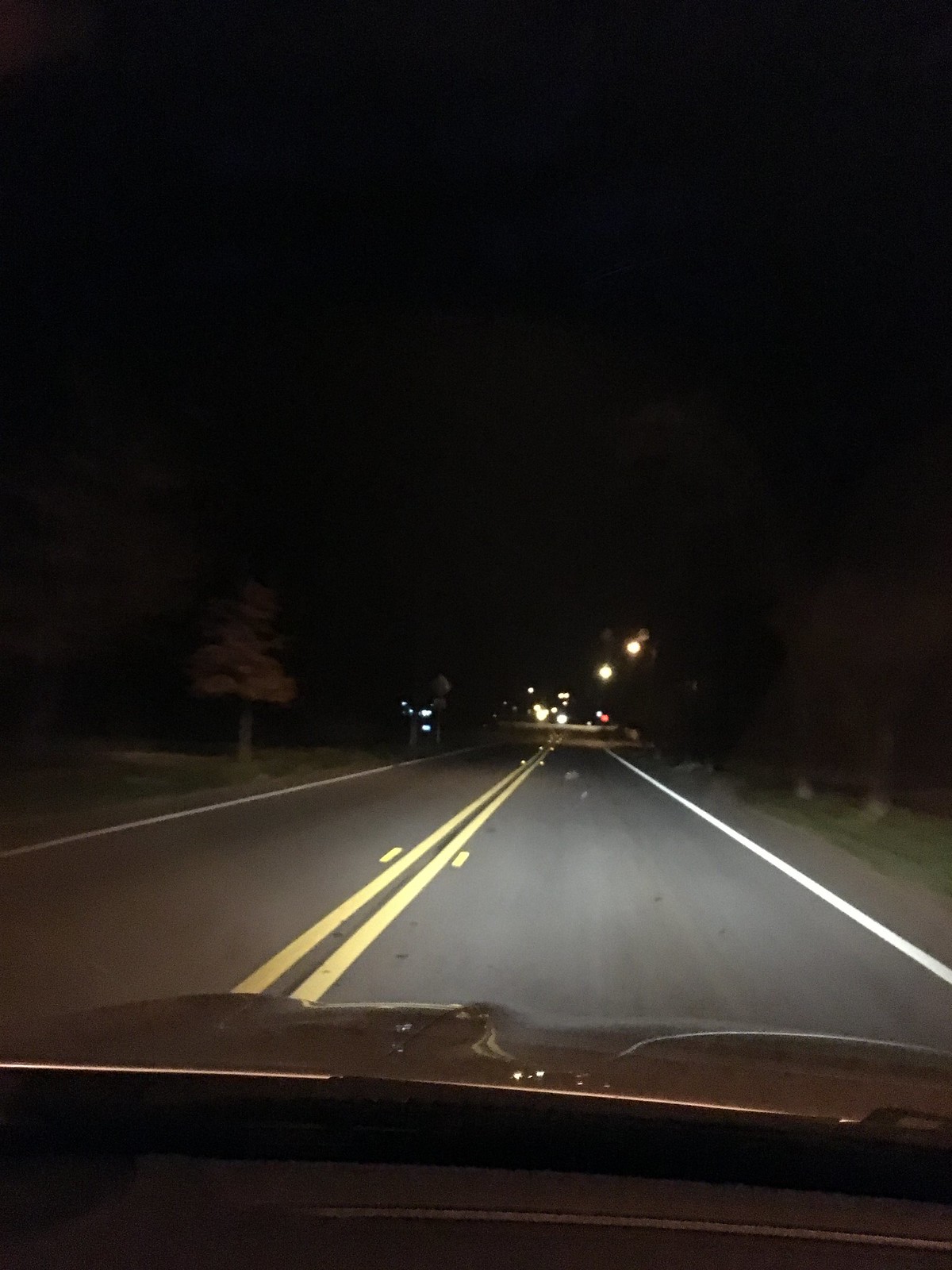The photograph captures an evening scene from inside a vehicle, looking out through the front windshield onto a dimly lit, single-lane road bordered by double yellow lines. The scene is enveloped in darkness, suggesting a night with minimal moonlight. Sparse street lights occasionally punctuate the otherwise shadowy roadway, revealing trees and grassy patches lining both sides. The lack of other vehicles on the road emphasizes the solitude of this suburban or rural setting, far removed from the constant illumination and bustle of an urban environment.